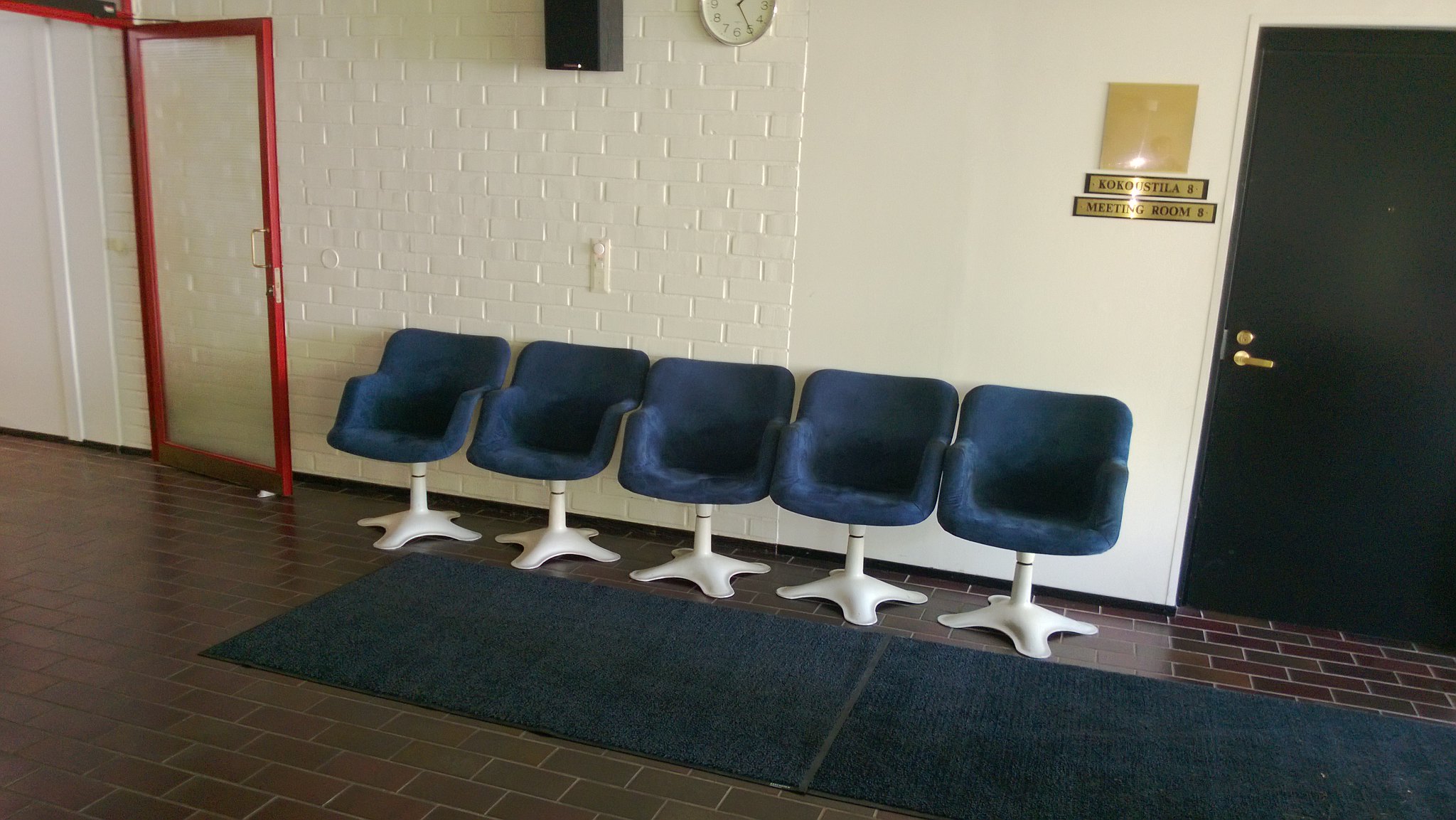The indoor photograph depicts a hallway, possibly within a school or office building. The walls are predominantly white, with a section of white-painted brick to the left and a white door labeled "Meeting Room." Two gold placards adorn the wall left of the door, which also features a gold lock and handle. Adjacent to the door is a row of five vintage blue chairs, aligned in a neat line. These chairs, appearing cushioned and comfortable, have a round and large mid-back design and are supported by white pedestal bases that extend into four feet. The chairs’ plush blue fabric contrasts with the dark brown tiled floor and a midnight blue carpet runner beneath them. Additional details in the hallway include a clock partially visible at the top middle of the image and a window or door on the left side of the frame, offering an exit from the hallway. Red-rimmed doorways and a solid black door further accentuate the space, adding to the retro ambiance reminiscent of the 60s or 70s.